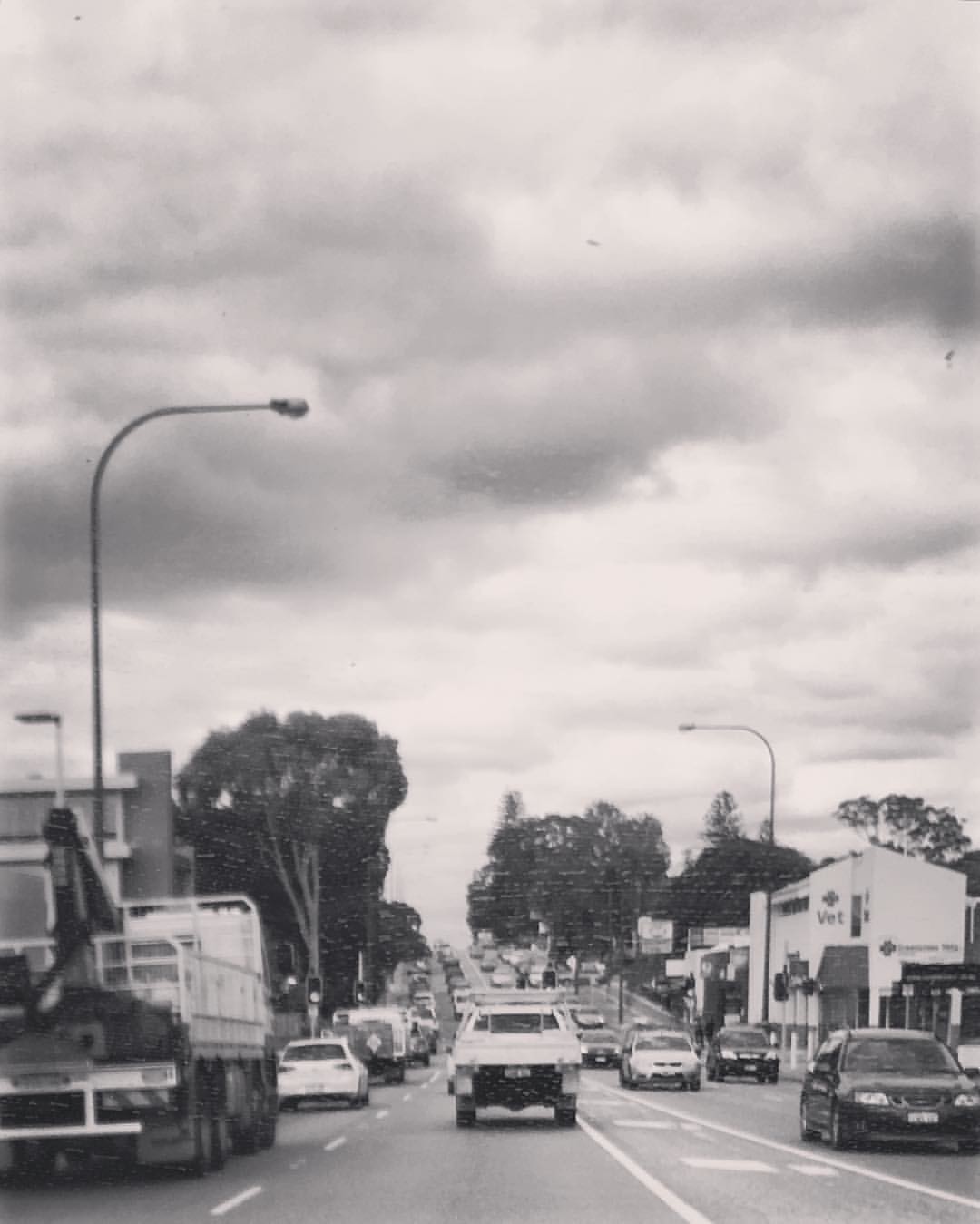This black and white photograph captures a bustling four-lane road in what appears to be a small town. The sky is heavily overcast, filled with dense clouds signaling imminent rain. To the left, a large truck with a truck bed and multiple wheels is visible, leading the flow of vehicles that proceed straight ahead while, on the right, a mix of white and black cars come toward the viewer. Traffic is organized by a median with dividing lines and some form of writing in between. Hanging street lamps and traffic lights punctuate the scene, suggesting a well-trafficked throughway. A white building labeled "Vet" with a prominent cross can be spotted on the right side of the road. In the distance, green trees line the street, adding a touch of nature to the urban setting, and hinting at the suburban outskirts of the town. There are also visible marks on the windshield, implying the photo was taken from inside a car, possibly through the streaks left by windshield wipers, further emphasizing the rainy setting.